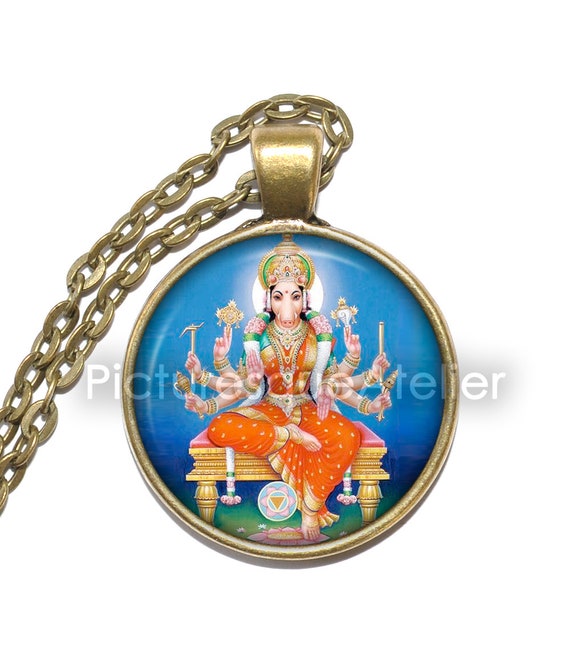This is a close-up angled image of an ornate gold pocket watch hanging from a gold chain. The pocket watch features a detailed illustration of a woman with six hands, three on each side, each holding a different item. She is depicted sitting on a gold bench with a red cushion, her right foot touching the ground and her left foot angled inward towards her thigh. The woman is adorned in a red dress with a gold crown accented in green, a distinct pig-shaped nose with tusks, and a dot between her eyes. Additionally, a moon is prominently positioned behind her head, and the background is filled with a deep blue hue. The pocket watch face also has subtly translucent lettering that reads "Pictures Q Atelier," giving it a unique, vintage appeal.